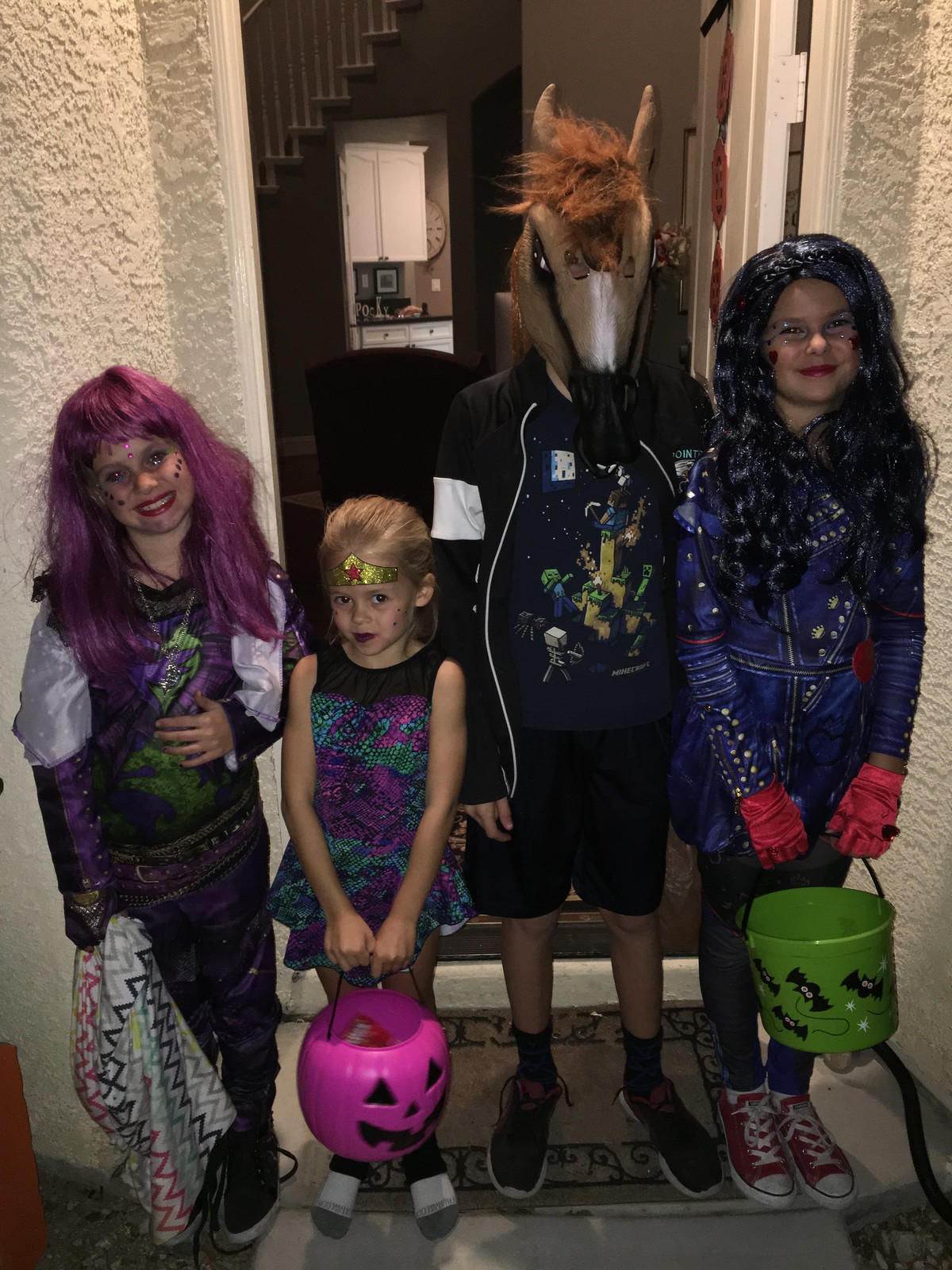In this vibrant Halloween scene set against a textured white wall and a stucco exterior, five individuals gather in front of a dark wooden door. The open doorway behind them reveals white cabinets, drawers, pictures, a clock, a staircase with a white railing against a beige wall, and a dark brown chair. 

On the far left stands a girl with long purple hair adorned with circular glitter pieces on her face. She wears pink lipstick and a shirt that transitions from white at the shoulders to purple at the wrists, covered in purple and green splotches, which match her pants. She holds a sack decorated with blue, red, and light gray triangles.

Next to her, a blonde-haired child dons a crown-like gold headpiece with a red star. She wears a purple and green frilled dress with dark green accents, complemented by glittery circles on her face. She clutches a hot pink pumpkin with black triangular features, filled with candy.

In the center, a person sports a black and white jacket over a Minecraft-themed shirt featuring characters like a skeleton, creepers, and a character in a cyan shirt. The individual wears a tan goat mask with white and black details.

To the right stands another individual in black shorts, a black shirt, black socks, black shoes, and a fluffy horse mask, holding nothing in particular.

Lastly, on the far right, a girl with long black curly hair is dressed in a dark blue suit with gold accents and red-pink gloves. She carries a green bucket adorned with black bats and white eyes.

The children, dressed in a variety of costumes and hairstyles, are ready for trick-or-treating, holding colorful Halloween buckets filled with candy as they stand on the doorstep.